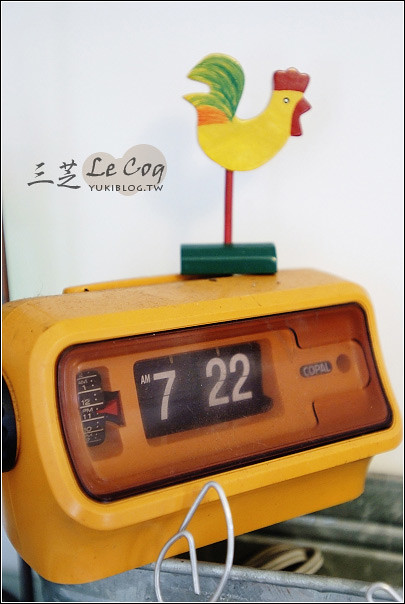The image depicts a vibrant, retro-style alarm clock, primarily yellow with orange accents, featuring a flip mechanism displaying the time as 7:22 a.m. The clock has a white numerical display on a black background and includes various dials, possibly for setting alarms or tuning a radio. Atop the clock, there rests a uniquely designed toy rooster, which might be a built-in feature associated with the alarm. The rooster has a yellow body, red comb, red beak, orange band, and green tail feathers, mounted on a red pole with a green base. The entire setup is placed on a metallic container. The background is stark white with the text "LeCog UBblog.tw" and some Chinese characters, potentially indicating the brand or source of the product.